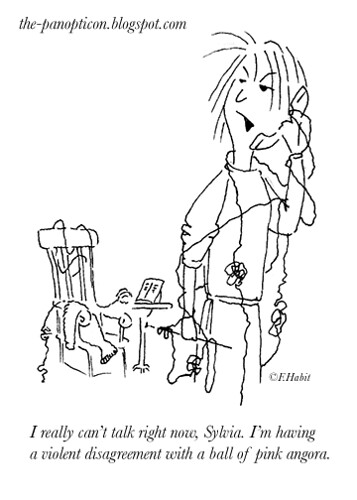The black-and-white sketch comic features a humorous scenario prominently titled "thepanopticon.blogspot.com" in black print on a white background. The focal point is a stick-figure woman with stringy hair, who is holding a phone to her left ear while entangled in yarn that appears to stretch from a table next to an old rocking chair in the background. Her right hand holds a knitting needle, emphasizing the tangled chaos of yarn around her. The caption humorously reads, "I really can't talk right now Sylvia, I'm having a violent disagreement with a ball of pink angora." Additionally, there is a signature by the artist noted as "F-H-A-B-I-T" in the lower right corner. The background details include a small chair draped with a sweater and a table holding a book, all adding to the quaint yet chaotic scene.